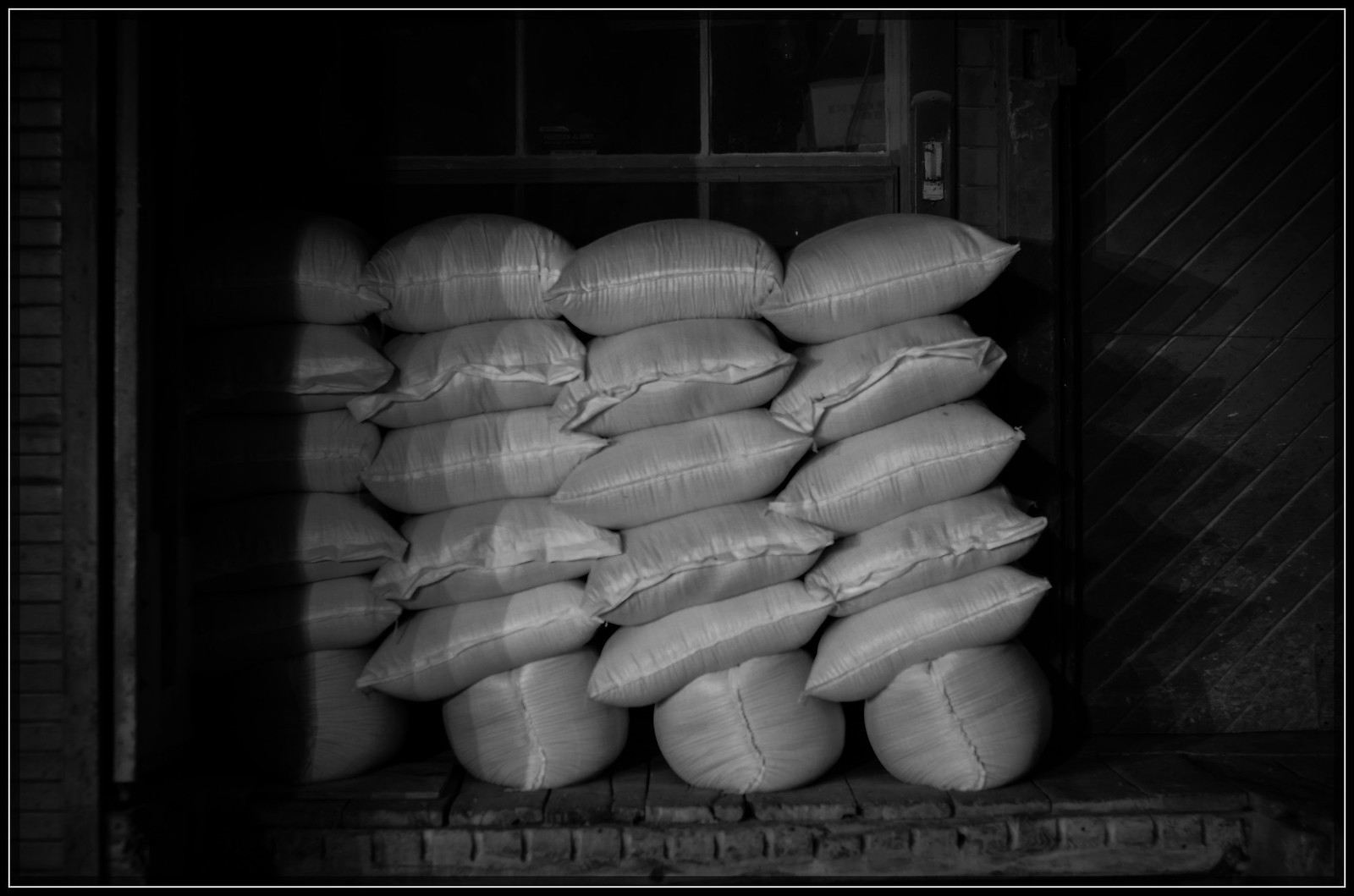This black and white photograph captures a striking scene of what appears to be rice bags or pillows stacked meticulously against the façade of a brick and mortar building, situated in front of a large window divided into several square panes. There are four stacks in total, with the bottom layer composed of bags or pillows standing on their sides, while additional layers of horizontally stacked bags create the subsequent rows. The stack furthest to the left is partially obscured by shadows, emphasizing the light and shadow contrast in the image. The brickwork, noted for its diagonal striped pattern at approximately a 40-degree angle, adds a textured backdrop, while the left side of the frame is noticeably dark, likely due to an external light source such as a streetlight influencing the image's illumination. The picture's details hint at an outdoor setting, possibly at night, with reflective light accentuating certain elements and casting distinct shadows to the right of the stacked items. The composition is a complex interplay of light, shadows, and textures, against a backdrop that includes elements such as a wooden shutter and a partially visible red wall.